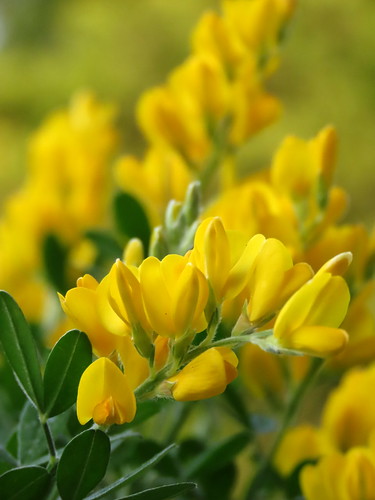In this close-up nature shot, a single small branch adorned with clusters of vibrant yellow flowers dominates the lower half of the vertical rectangular frame. Each flower sits gracefully on a much lighter green stalk compared to the darker oval green leaves present at the bottom left of the image. The intricate details of the heart-shaped petals and the whitish center stalk are captured sharply. Beyond this primary branch, the background transitions into a soft blur, creating a Bokeh effect that suggests a field filled with similar yellow flowers. This blurred backdrop not only emphasizes the main subject but also subtly showcases overlapping green twigs and additional clumps of yellow blooms fading into a serene, indistinct green expanse.